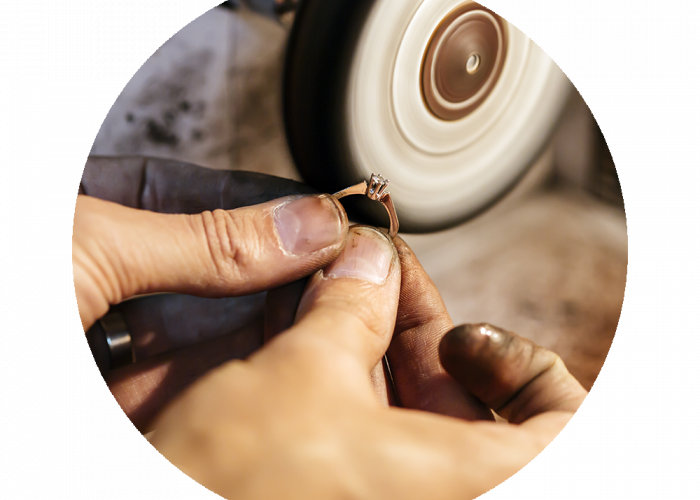In a round-framed image featuring a jeweler's workspace, a pair of hands diligently works on polishing a diamond ring. The left-hand thumb, visible from the middle left side, presses against the edge of the gold ring adorned with a diamond centerpiece. The thumb is positioned over a black material, possibly part of the jeweler's tool setup. Simultaneously, the right hand enters from the bottom, with its thumb and middle finger steadily gripping the ring. The forefinger, bent and further down, supports the process. Both hands appear worn and smudged from a day's work, indicating the craftsmanship involved. 

In the top right of the image, slightly out of focus, is a large, spinning polishing wheel. The wheel, black on the outside, white on the inside, and brown in the center, suggests the ring is being polished rather than cut or ground. The background is blurred, with a light grey hue, drawing attention to the intricacy of the jeweler's task. The subtle details and precise hand positioning capture the intimate and careful nature of working with fine jewelry.